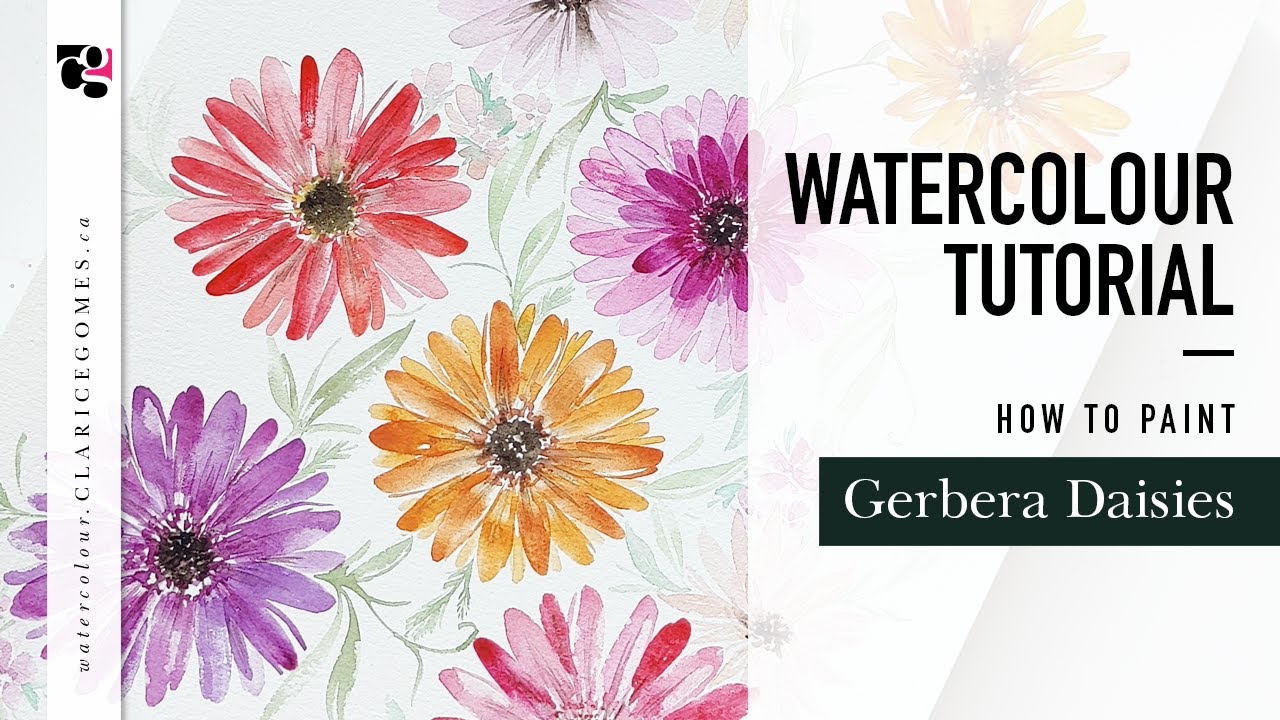This horizontal, rectangular image features a white background with an illustrated array of colorful flowers, including hues of purple, pink, orange, yellow, red, and fuchsia, accompanied by green leaves, all painted in watercolor. The left side showcases the artist's work with a variety of Gerbera daisies, meticulously rendered to highlight their vibrant colors. On the far left, the text reads "watercolor.clarissegomes.ca." Meanwhile, the right side of the image contains a vertical white border displaying the instructional text in sequential green and black letters: "watercolor tutorial," "how to paint," and "Gerbera daisies." The cover is designed to resemble the first page of a watercolor tutorial book by Clarisse Gomez, offering a detailed guide on painting these beautiful flowers.